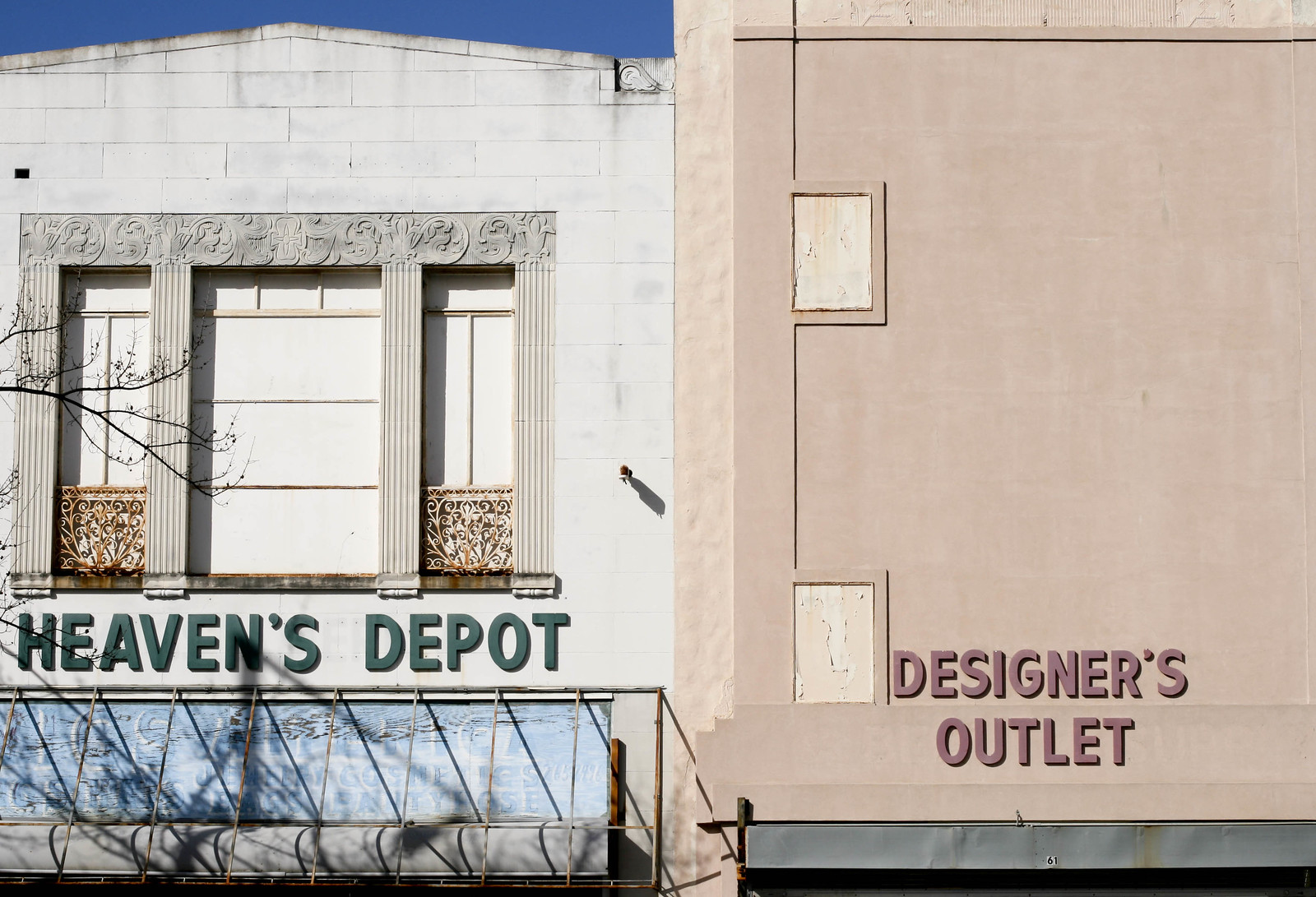The color photograph showcases the frontage of two adjacent buildings taken from a detailed perspective. On the left is an older white sandstone building from the early 1900s, identifiable by its weathered appearance and white brick facade with off-white columns adorned with a grey pattern. The top of this building features a peaked roof and three large windows on the second floor, outlined by stone pillars and topped with a decorated plinth. Gold scrollwork embellishes the bottom of the two side windows, though these are boarded up with white boards. Below the windows is a dark green sign reading "Heaven's Depot," positioned above a rolled-up pale blue awning, and a blue and grey tarp secured by square metal meshing. Adjacent to it, on the right, stands a beige building with a flat facade featuring a deeper sand inset in its plaster outline. It bears a grey banner near the bottom with "Designer's Outlet" written in light purple lettering. The upper portion of this building includes two rectangular insets harmonizing with the plaster's color scheme. The photograph also captures a portion of dark blue sky above the roof of Heaven's Depot, and notably, there are no people, animals, plants, or motor vehicles in the scene.